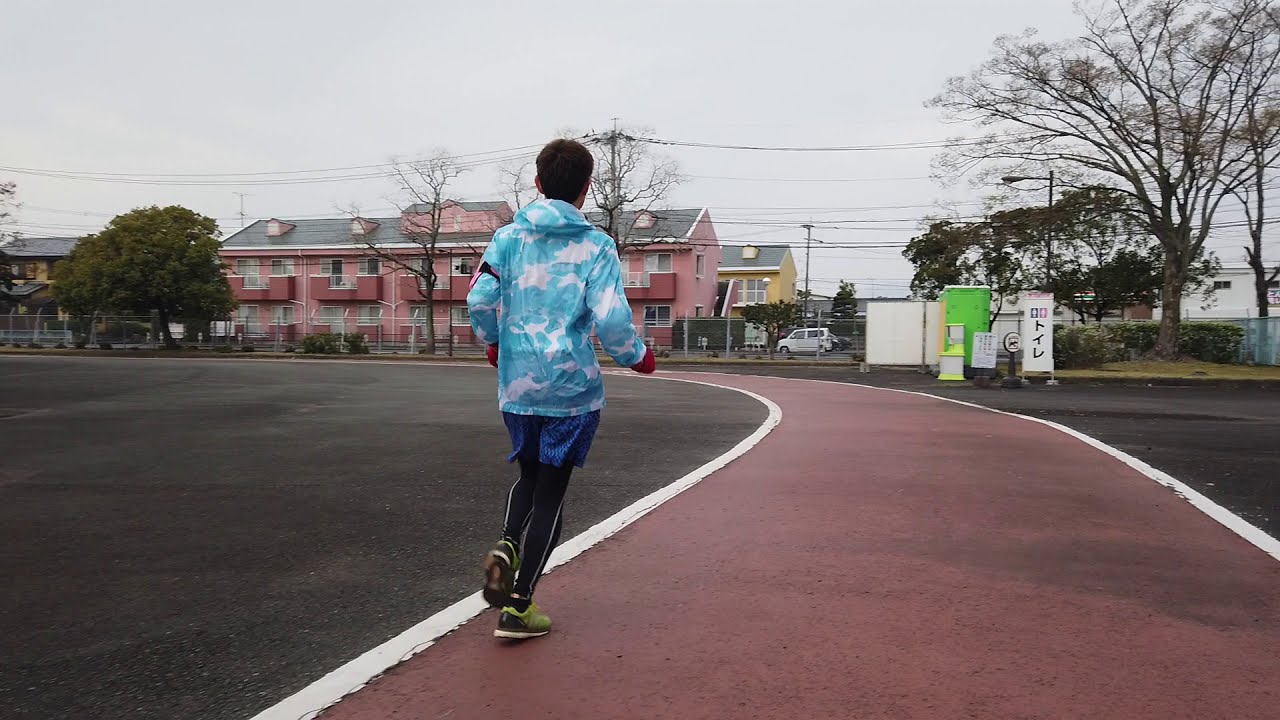The photo captures the rear view of a young boy running slightly off-center to the left on a red track outlined with white lines, nestled within a larger asphalt area. He has dark brown hair and is dressed in a blue sweatshirt adorned with white, cloud-like patches, reminiscent of a sky. Complementing his outfit, he sports blue shorts over black leggings, red gloves, and black and green running shoes. His pose captures the motion of running, with his right foot on the ground and his left foot raised.

In the background, there's a mix of urban and natural elements. A white sign with illegible foreign text, likely Japanese, is visible. Behind the sign stands a large two-story apartment building with gray roofs, and what appear to be multiple stacked units viewed from the back, suggesting residential condos. Adjacent to this building, there is a small green structure, resembling a porta potty, along with a pink and orange building in the vicinity, adding more color diversity to the scene. Enveloping these structures is a scattering of trees, and over the image, electrical power lines hang visibly against a gray sky. The environment suggests a serene, suburban area with a track dedicated to sports activities.